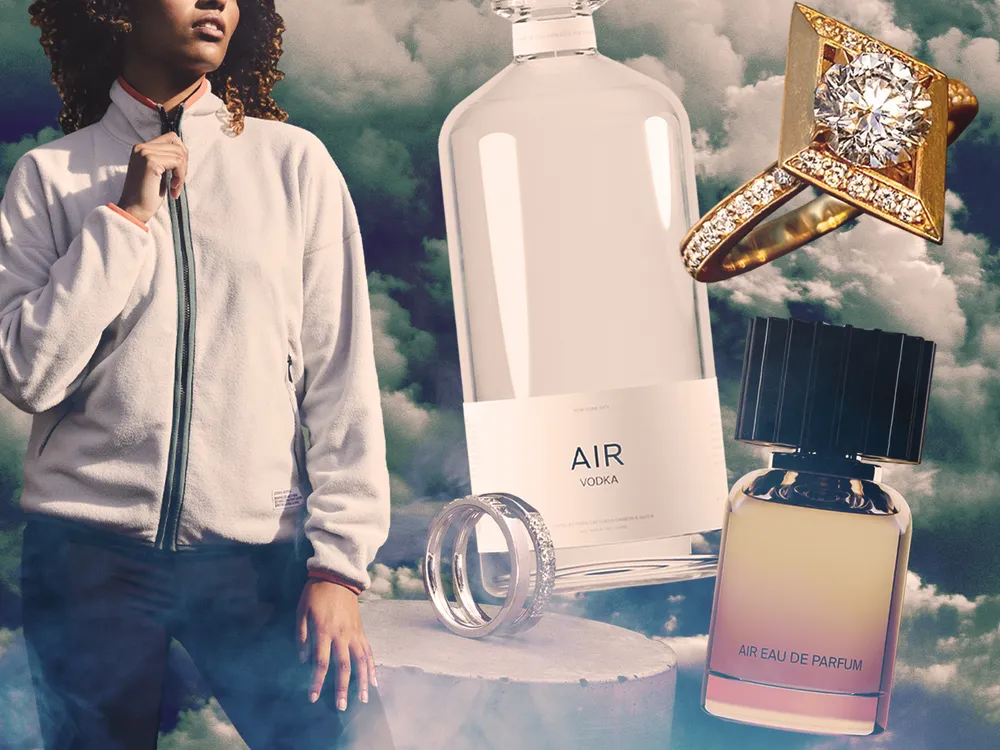This image resembles an advertisement with an eclectic collage of items set against a backdrop of clouds. To the far left, a woman wearing a white fleece jacket with a black zipper and blue pants is positioned. Her curly brown hair cascades around her face, which is partially obscured, showing only from her nose down to her thighs. Her right hand grasps the top of the zipper near her neck while her left hand rests on her thigh.

To her immediate right, a bottle labeled "Air Vodka" is prominently displayed. The transparent, glass bottle with a screw-off top appears filled with a clear liquid. Below this bottle, two intertwined wedding rings sit atop a concrete pedestal; these rings are similar in design but vary in their silver hues, adorned with diamonds.

Further to the right, a lavish wedding band with gold plating and encrusted with diamonds on its band boasts a large, circular diamond centerpiece. Below this opulent ring, a perfume bottle labeled "Air Eau de Parfum" can be seen. The bottle, tinted brown with a black oversized cap, is described as having a watery brown perfume within.

Throughout the image, no distinct borders separate the items, which enhance the collage's assorted and imaginative feel, suggesting the arrangement may be digitally created to capture attention and convey luxury through the juxtaposition of the products.